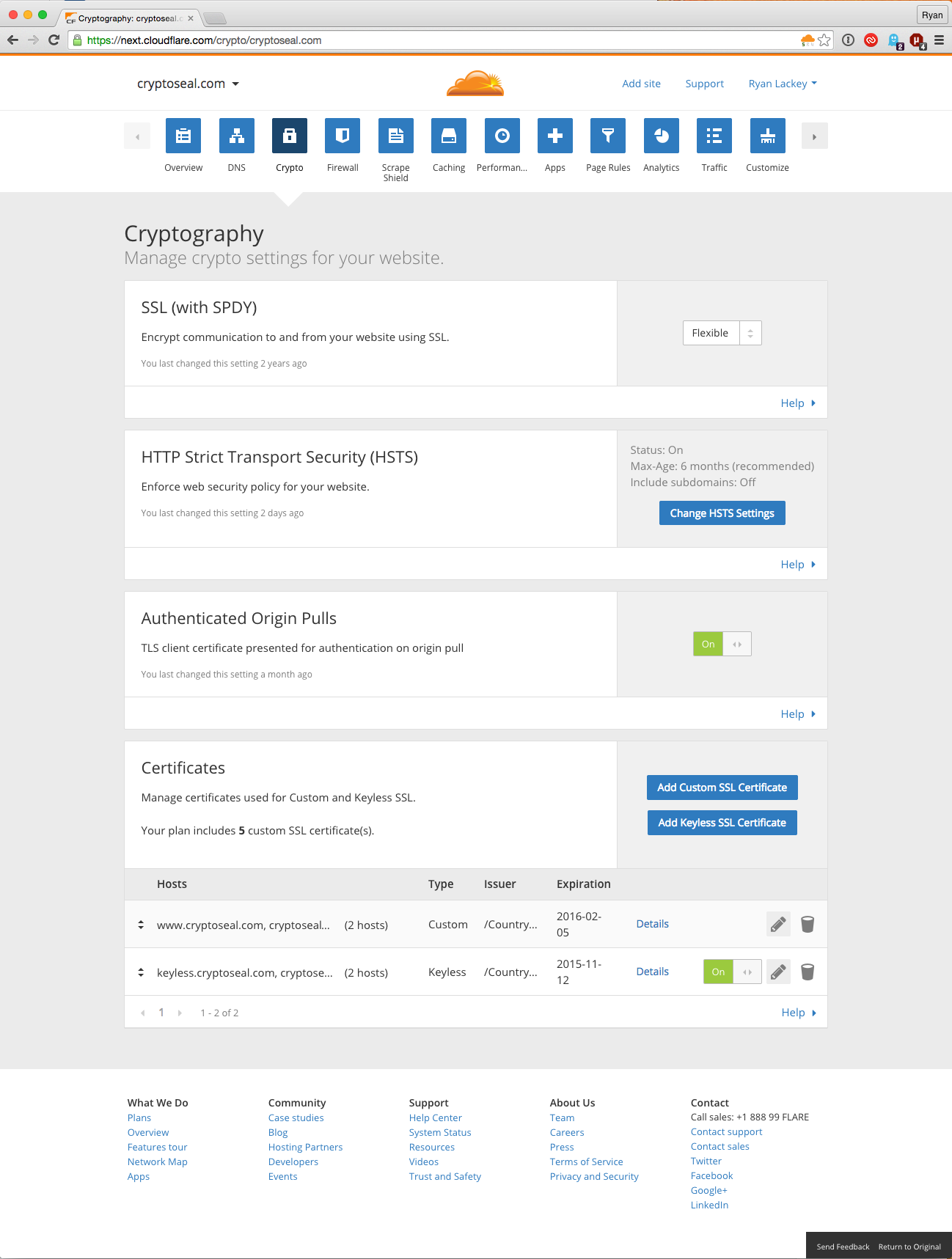Screenshot of a website management interface featuring various categories in a top navigation bar located centrally. The categories listed are: Overview, DNS, Crypto, Firewall, Scrape Shield, Caching, Performance, Apps, Page Rules, Analytics, Traffic, and Customize. Below this navigation bar, on the left side, there is a section titled "Cryptography" with a subtitle that reads "Manage crypto settings for your website." The options available in this section include SSL with SVDY, HTTP Script Transport Security (HSTS), Authenticated Origin Pools, and Certificates. At the bottom of the interface, there are two websites listed under a heading that indicates "Two Hosts" to the right.